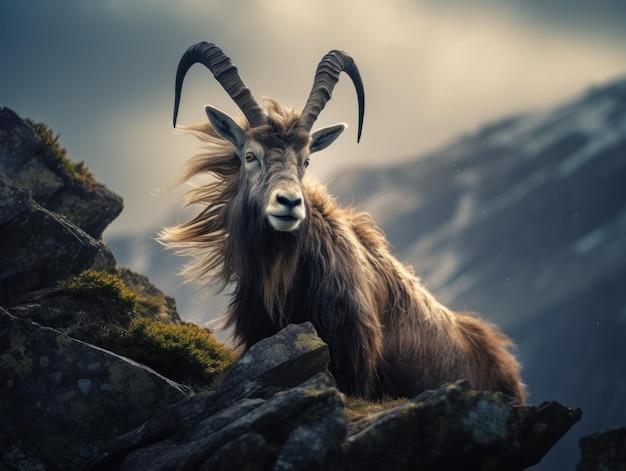The image features a striking mountain goat perched on rugged cliffs. The goat, with its extravagant, curved black horns that sweep back towards its body, is the main focal point of the photograph. Its shaggy, golden-brown fur, which appears almost illuminated by the sun, creates a glowing effect. The animal's thick, flowing hair is notably long at the neck, blowing gently to the left. The goat's body, including a lighter brown patch on its midsection, stands out against the jagged, dark gray rocks adorned with green vegetation and moss. The scene is set against a blurred, multi-colored background where hues of dark blue transition to patches of light, likely reflecting sunlight through clouds. The rugged terrain features rocks taller on the left side and elevating to the goat's level on the right, enhancing the sense of adventure and natural beauty.